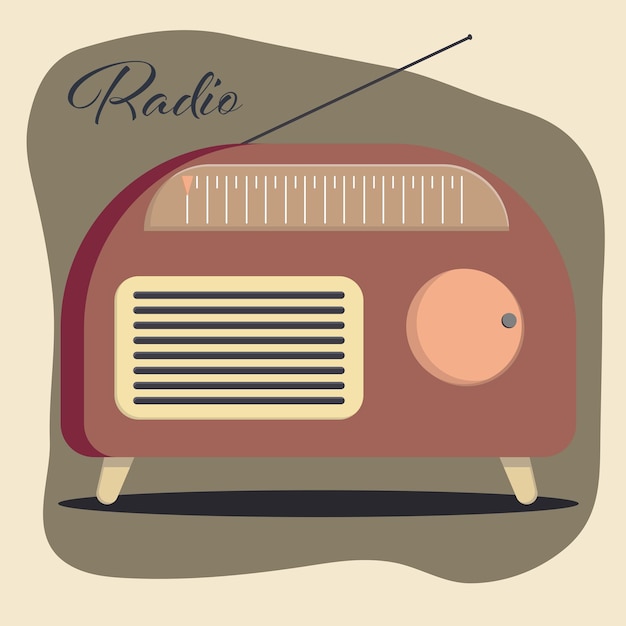The image is a detailed graphic illustration of a vintage radio, positioned centrally against a muted green and beige background. The radio itself has a curved rectangular shape, predominantly brown in color. It stands on two yellow legs and casts an elliptical shadow beneath. An orange volume knob is situated on the right side, while a rectangular, rounded speaker with horizontal blue lines occupies the left side. Above the speaker is the calibration for radio signals. A black antenna extends diagonally from the top left of the radio. In the top left corner of the image, the word "Radio" is written in a blue script font, enhancing the vintage aesthetic.